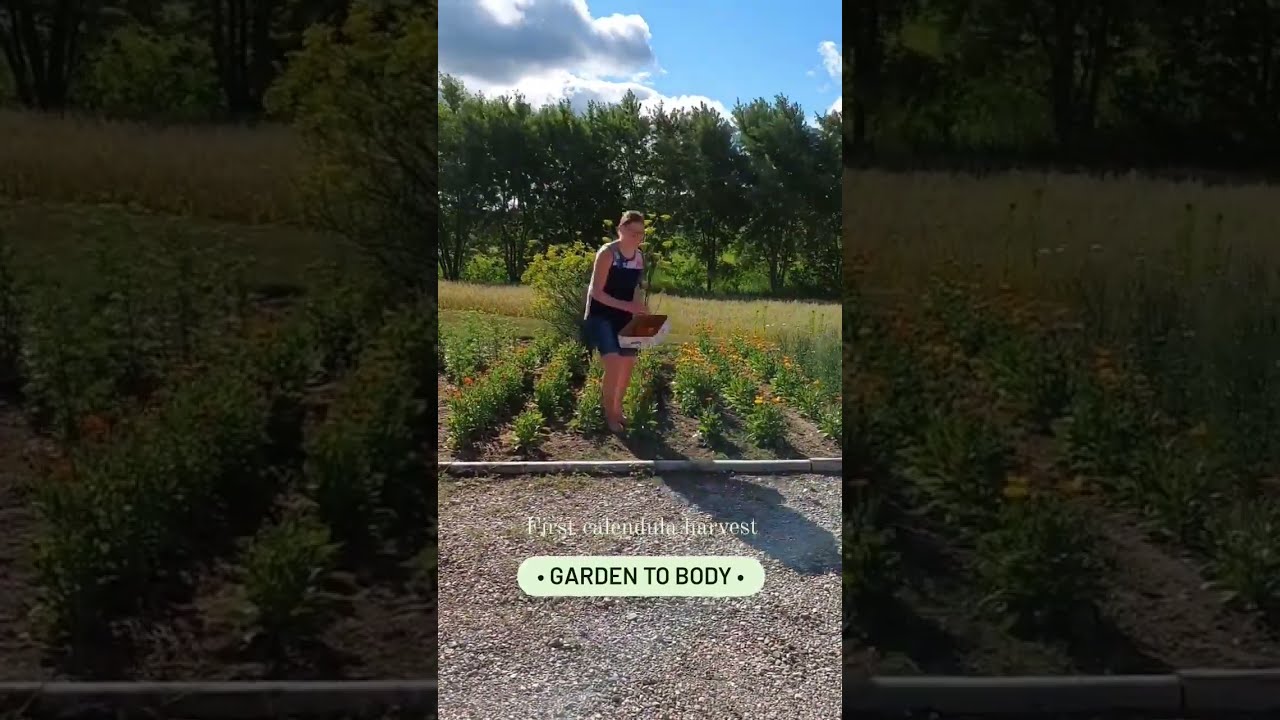The photograph depicts a garden scene with a central focus on a young Caucasian woman wearing a blue skirt and black top, holding a small white or cardboard box. The image is segmented into three parts, with the left and right thirds zoomed in and faded to half the lighting of the center. The garden occupies a square bed filled with about eight or nine rows of short green plants, surrounded by wood chips, pebbles, and rocks. The scene is set during the daytime under a partly cloudy sky with the top 20% of the image showcasing trees in full summer bloom. Behind the woman, there's a field of tall grass, bushes, and very tall dark green trees. The woman is positioned slightly to the four o'clock direction, appearing to interact with the contents of her box either by collecting or planting seeds. At the bottom of the photo, text in off-white writing reads "First calendar harvest," with "garden to body" underneath.